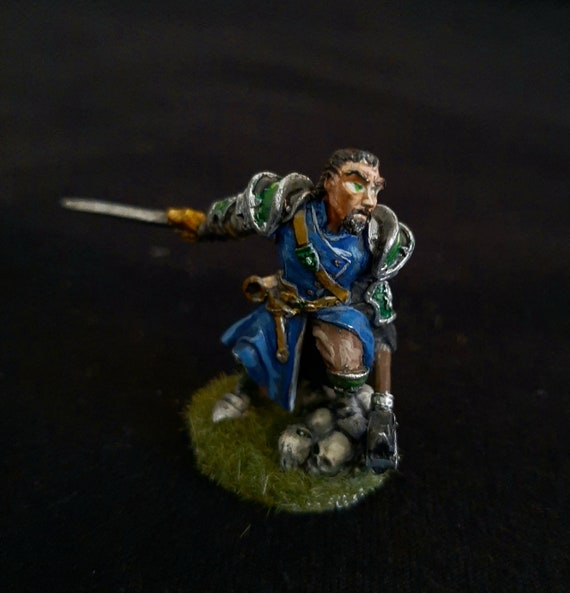In the center of a black background, a small figurine, approximately two inches tall, stands prominently. The character appears to be a historical fighter, possibly a knight or jester, adorned in a blue battle coat with armor on the shoulders. His detailed attire includes a blue overcoat and metal plates over the top of his shoes. The figurine depicts a white man with brown hair and a goatee, wielding a gray sword in his right hand, poised as if ready for battle. In his left hand, he holds a club with a wooden shaft and a black head, adding to his warrior-like appearance. Surrounding his feet are four or five human skulls, and he stands on a small, round patch of grass, about two inches in diameter. The image has a blurred effect around the edges, drawing focus to the intricately crafted figure in the center.